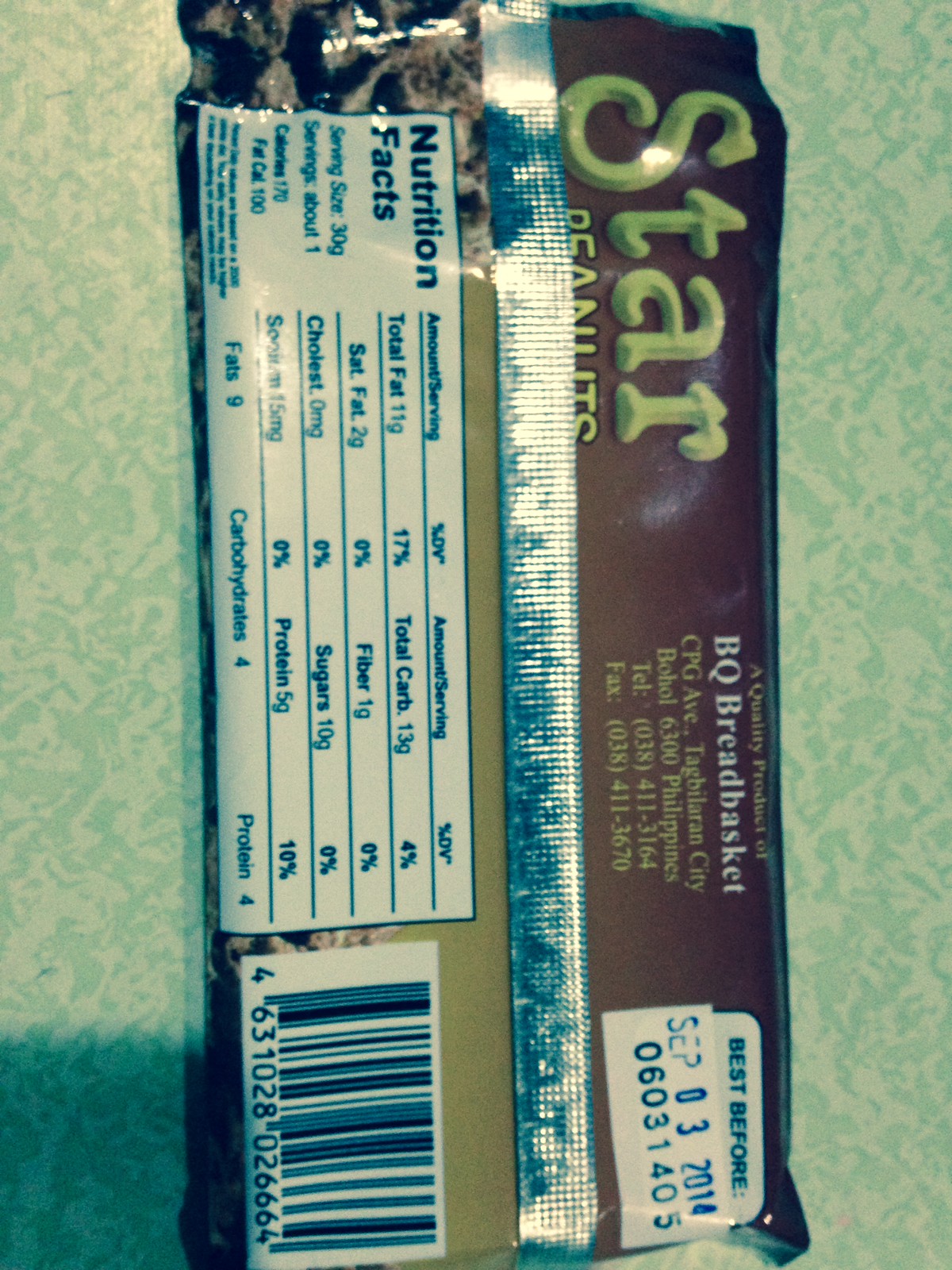The image displays a pack of peanuts, possibly resembling a candy bar, tilted sideways against a green, two-tone background with a subtle floral pattern reminiscent of wallpaper. The brown wrapper features several key details: 

- In the top left corner, large green letters spell out "STAR," with "peanuts" written in smaller font below it. 
- To the right, in a light green font, it states "a quality product of" followed by "BQ Bread Basket" in white. Additional information in green includes "CPG Avenue, Tagbilaran City, Bohol 6300 Philippines, Telephone 038411-3164, Fax 038411-3670."
- There is a white box carrying the text "Best Before" in blue, the contents of which are stamped with September 03, 2014, in the same blue hue, accompanied by the number "06031405."
- Centered on the wrapper is a section with silver foil.
- Below this is a white box displaying nutritional facts: Serving size of 30 grams, approximately 1 serving, 170 calories (100 from fat), 11 grams of total fat, 2 grams saturated fat, 0 milligrams cholesterol, 15 milligrams sodium, 9 grams total fat, 4 grams carbohydrates, and 4 grams protein.
- Adjacent to the nutritional facts is a barcode on a beige background, numbered “4631101028026664.”

In the upper left corner, a faint, unclear image of nuts can be seen. The green background of the overall image enhances the contrast, featuring white floral designs, creating a formica-like texture.